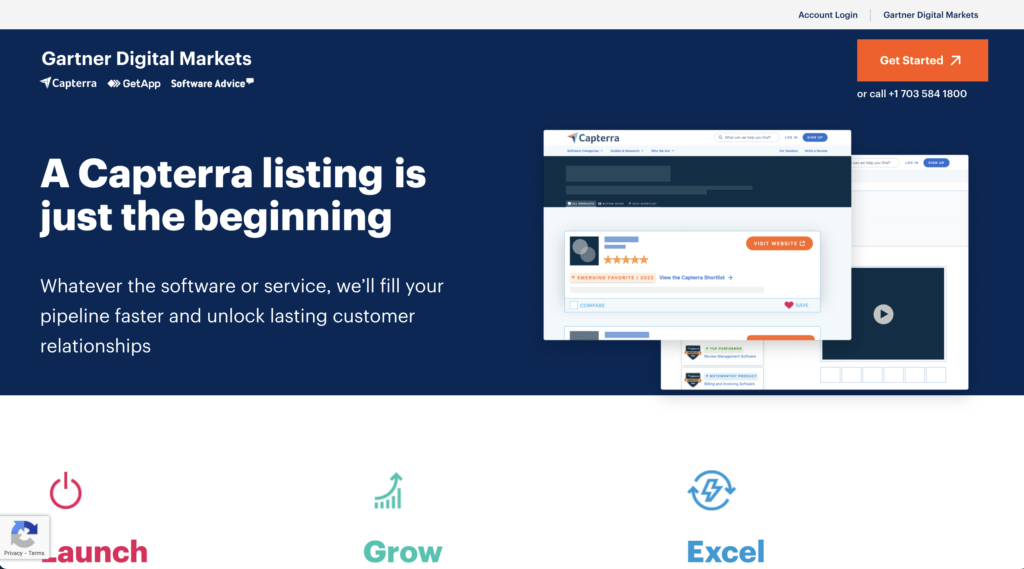The image depicts a webpage for Gartner Digital Markets, a company name prominently displayed at the top left of the page in white text. A gray navigation bar spans the top of the site, with blue text links for "Account Login" and "Gartner Digital Markets" located on the upper right-hand side.

Below the navigation bar is a large blue rectangle, occupying roughly a quarter of the image. Inside this rectangle, in the upper left-hand corner, "Gartner Digital Markets" is written in prominent white text. Directly beneath this are three smaller white texts: "Capterra," "Get App," and "Software Advice."

The main section of the blue rectangle features bold white text stating, "A Capterra listing is just the beginning," indicating the primary focus of the page. Following this header is smaller text explaining that the software or service will fill the pipeline faster and help unlock lasting customer relationships. To the right of this text are two smaller screenshots showcasing their webpage interface.

In the upper right corner of the blue rectangle, there is a "Get Started" button, and below it, a customer service phone number is displayed. At the bottom of this blue section, from left to right, are three buttons labeled "Launch," "Grow," and "Excel."